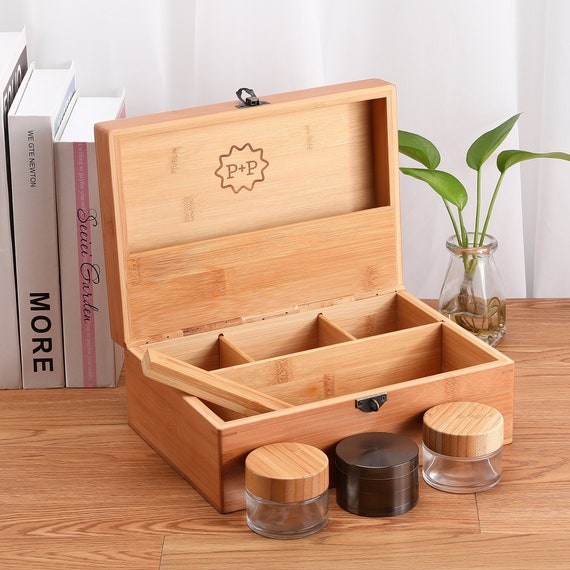This color photograph features a light beige wooden box sitting on a light wood grain table with a white wall in the background. The box, which has its lid open, reveals the interior compartments: three small ones at the top and one long compartment at the bottom. A black metal clasp secures the lid when closed. Inside the lid, there is a decorative circular emblem with the letters "P + P" at the center. 

In front of the box are three small jars: the two on the sides are round glass jars with matching wooden lids, while the jar in the center is black, possibly made of metal. A wooden stick is partially visible, sticking out from one of the box's compartments.

To the left of the box, there are three stacked books. The titles are mostly unreadable, but the middle one has the word "MORE" clearly printed on its spine. To the right, a clear vase with water holds a green plant with four leaves.

This setting, reminiscent of a neatly arranged display, could be intended for showcasing the wooden box and its accompanying jars, which might be used for storing items like spices.